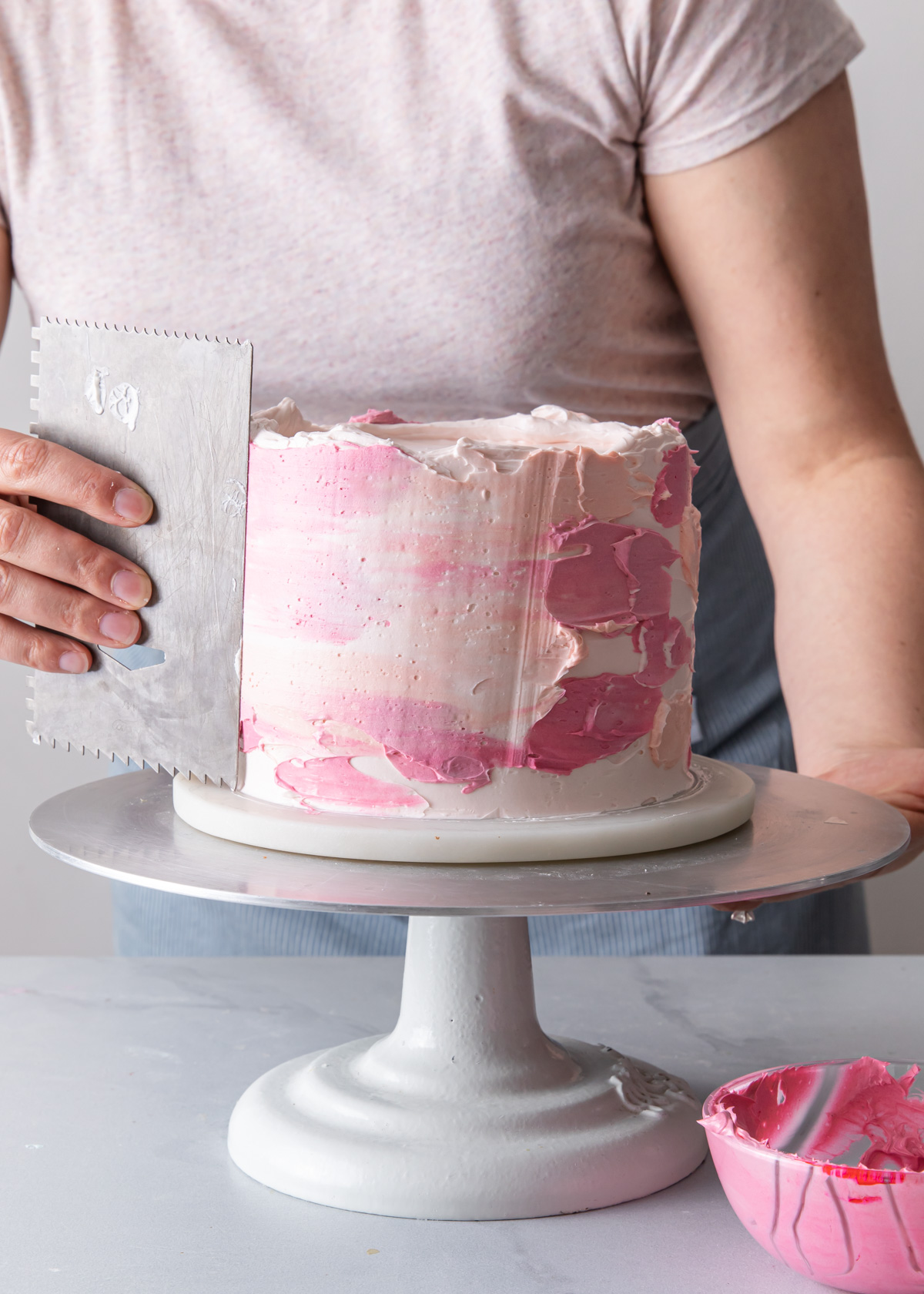In the image, we see a woman in the process of frosting a cake, captured from just above her shoulders to her knees. She is wearing a pink t-shirt paired with a blue skirt. The cake rests on a silver-colored platter with a white legged base, sitting on a white marble countertop with thin gray streaks. The cake itself is round and tall, with its sides being smoothed out by a metal spatula held in her right hand. Her left hand steadies the cake by holding the base. The frosting on the cake is primarily white with peach and pink splotches. In the bottom right corner, there is a bowl containing pink icing. The woman’s careful attention and the detailed cake-decorating process indicate she is meticulously working to finish the cake's frosting.